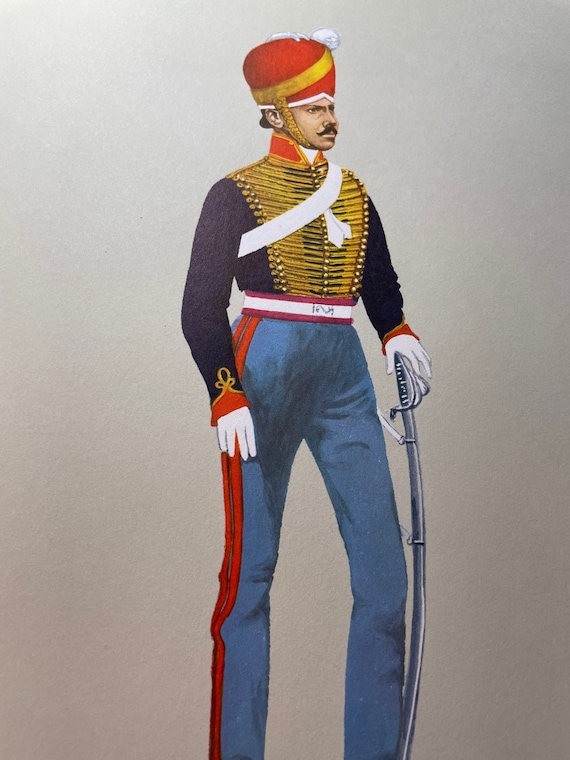This detailed drawing presents a full-length portrait of an Indian military officer, standing centralized against a gray background. The officer is depicted in an elaborate traditional uniform, featuring a distinctive red turban with a gold band, gold chinstrap, and adorned with a white pompon on top. His upper body is dressed in a blue military jacket, accented with intricate gold braiding and a striking red collar. A white sash crosses his chest, adding to the regal appearance.

He wears blue trousers, notable for the two red stripes running along the sides, paired with white gloves on both hands. The officer's posture is commanding, with one hand resting on a traditional silver saber pointed downwards toward the ground. The white belt around his waist, edged with red stripes, complements the overall color coordination of his sophisticated uniform. Despite the elongated representation of his legs, the image captures the essence of a dignified and authoritative military figure, rich in cultural and historical detail.